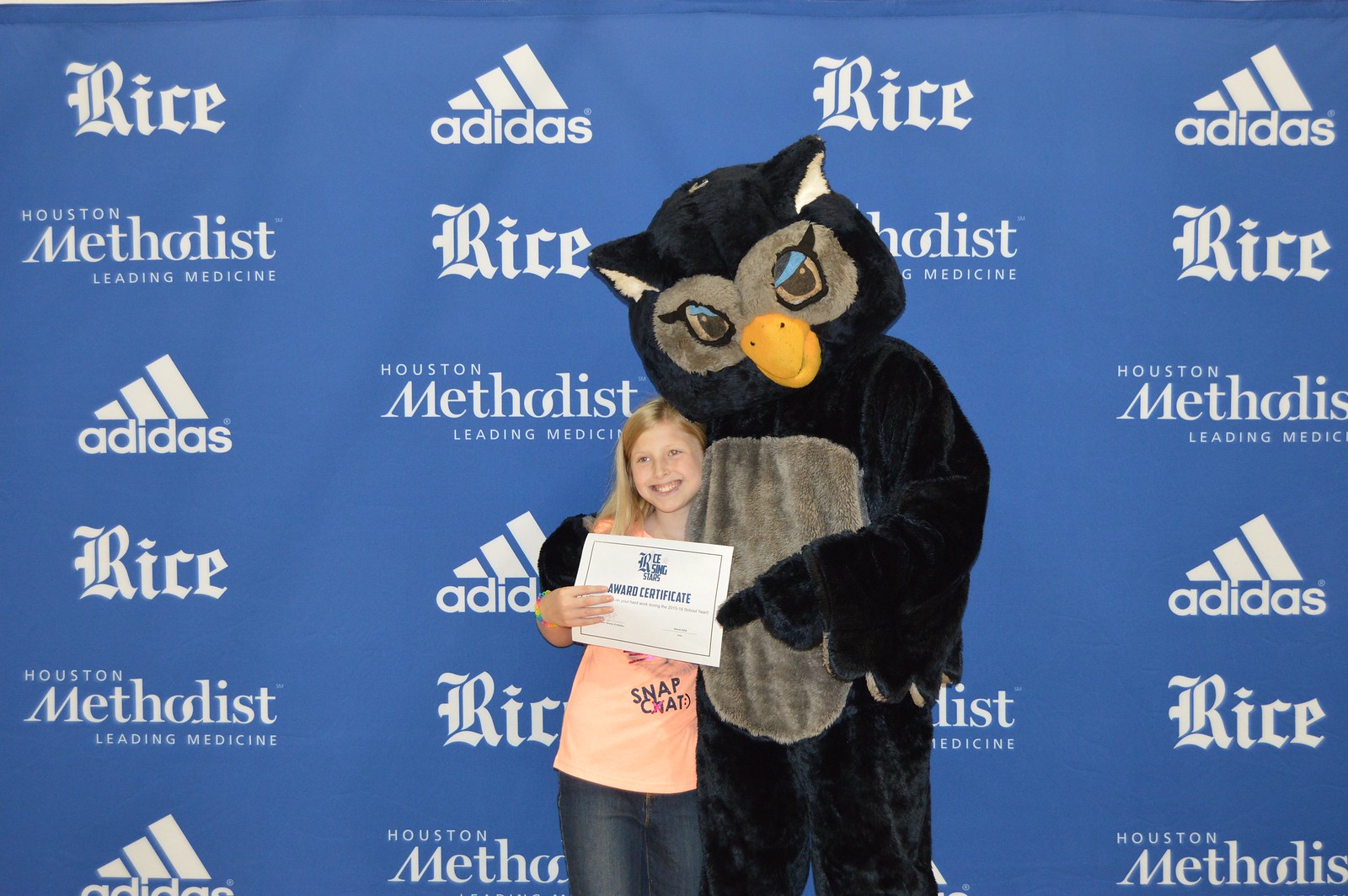A vibrant color photograph captures a young girl, around 11 or 12 years old, with blonde hair, smiling brightly as she stands next to a large black owl costume character. The owl, adorned with blue eyes, a yellow beak, and a gray and white chest patch, has its left arm extended forward with stubby fingers and its right arm affectionately wrapped around the girl. The owl also boasts white interiors in its black ears and stands at least a foot taller than the girl. The girl is wearing a light pink t-shirt with "Snapchat" emblazoned on it, paired with blue jeans, and she proudly holds a white award certificate with blue text. They pose in front of an expansive blue banner covered in repeating white text that reads “Rice,” “Adidas,” “Houston Methodist,” and “leading medicine,” indicating the backdrop ties to Rice University in Houston.